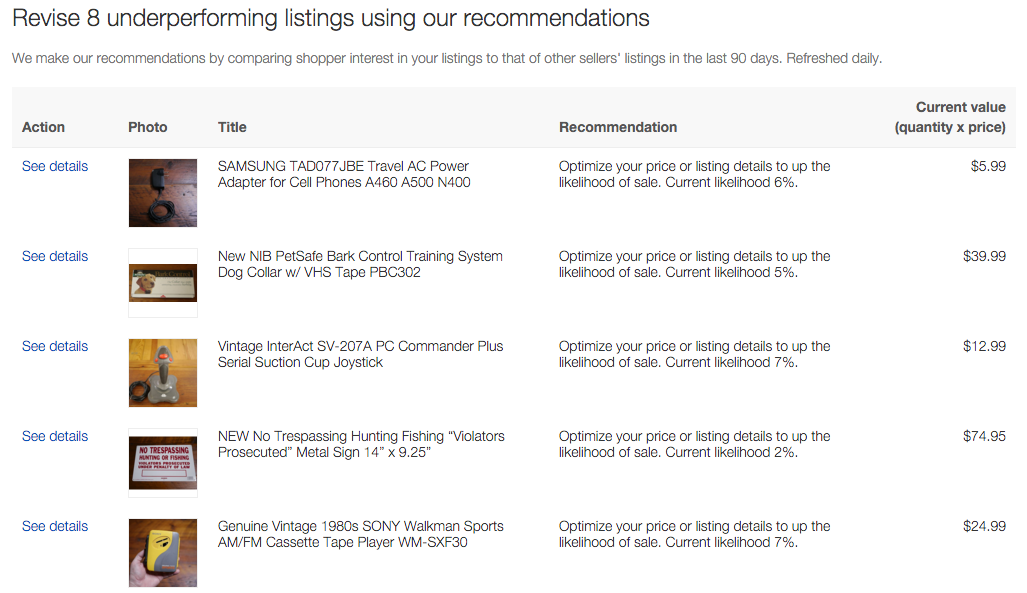The image displays a dashboard with a headline reading, "Revise 8 underperforming listings using our recommendations." Below the headline, there's an explanatory note in grey text that says, "We make our recommendations by comparing shopper interest in your listings to that of other sellers' listings in the last 90 days, refreshed daily."

Underneath the explanatory note, there’s a chart with five columns labeled: Action, Photo, Title, Recommendation, and Current Value (Quantity x Price). In the Action column, each listing has a blue link labeled "See details."

The listings start with an image of each item. The first item is a Samsung TAD077JBE travel AC power adapter for cell phones, including specific model numbers. The recommendation for this item suggests, "Optimize your sale price or listing details to increase the likelihood of sale. Current likelihood is 6%." Its current value is marked as $5.99.

The second item is a "New in Box Pet Safe Bark Control Training System Dog Collar with VHS Tape."

The third item is a "Vintage Interact CV-207A PC Commander Plus Serial Suction Cup Joystick."

The fourth item is a sign reading "No Trespassing, Hunting, Fishing."

Finally, the fifth item is a "Genuine Vintage 1980s Sony Walkman."

Each recommendation aims to improve the performance of these listings based on competitive shopper interest over the past 90 days.